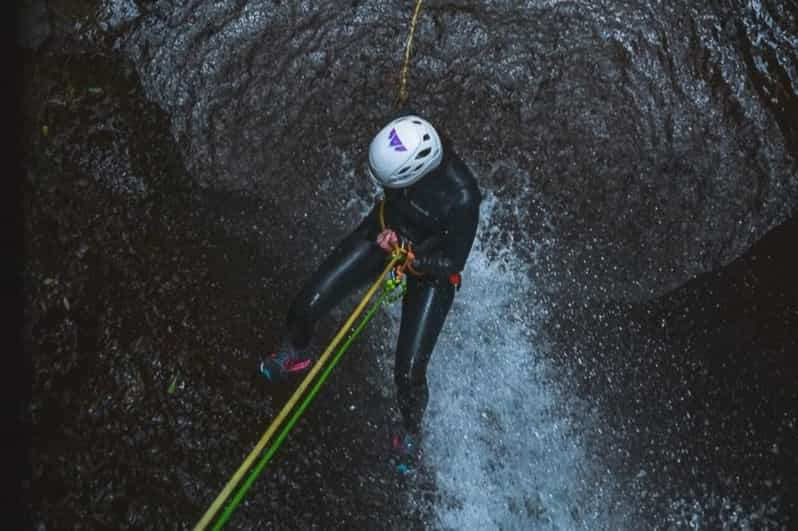This photograph offers a dramatic bird's-eye view of a climber meticulously rappelling down the vertical side of a dark, deep cave adjacent to a powerful waterfall. The climber, wearing a full black wetsuit and a white safety helmet, is seen holding onto vibrant green and yellow ropes as they make their descent. Their colorful shoes, adorned with pink and blue lines, are poised next to the cascading water that flows vigorously down the cavern's rough, gray and brown walls. The water splashes just beneath them, emphasizing the depth and intensity of the descent. The climber's body is positioned carefully, looking downwards, navigating the descent with precision as the waterfall rushes alongside them into the pool below.